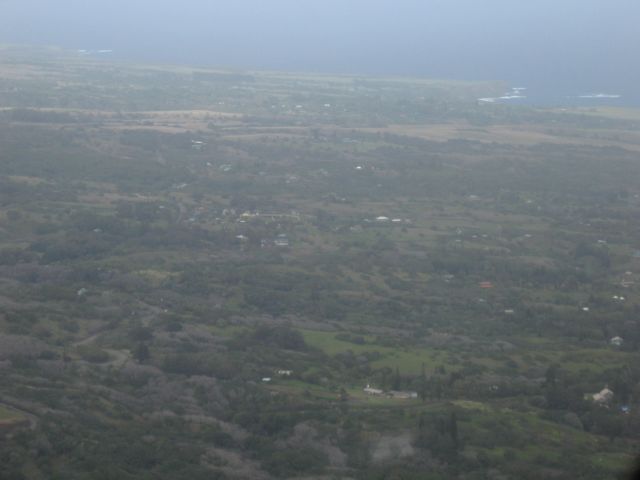The aerial photograph, likely taken from a helicopter, plane, or drone, captures a rural shoreline region shrouded in a light mist or fog, obscuring some details. The top portion of the image features a body of water with white wave crests breaking against the cliffs. The land below is hilly and predominantly green, dotted with scattered homes, some of which are white with black roofs. The terrain includes grassy areas, fields, and patches of trees and bushes. The combination of open land and vegetation suggests a mix of farmland and natural landscape. The foggy atmosphere adds a soft, diffused light to the scene, making it appear tranquil and somewhat ethereal.